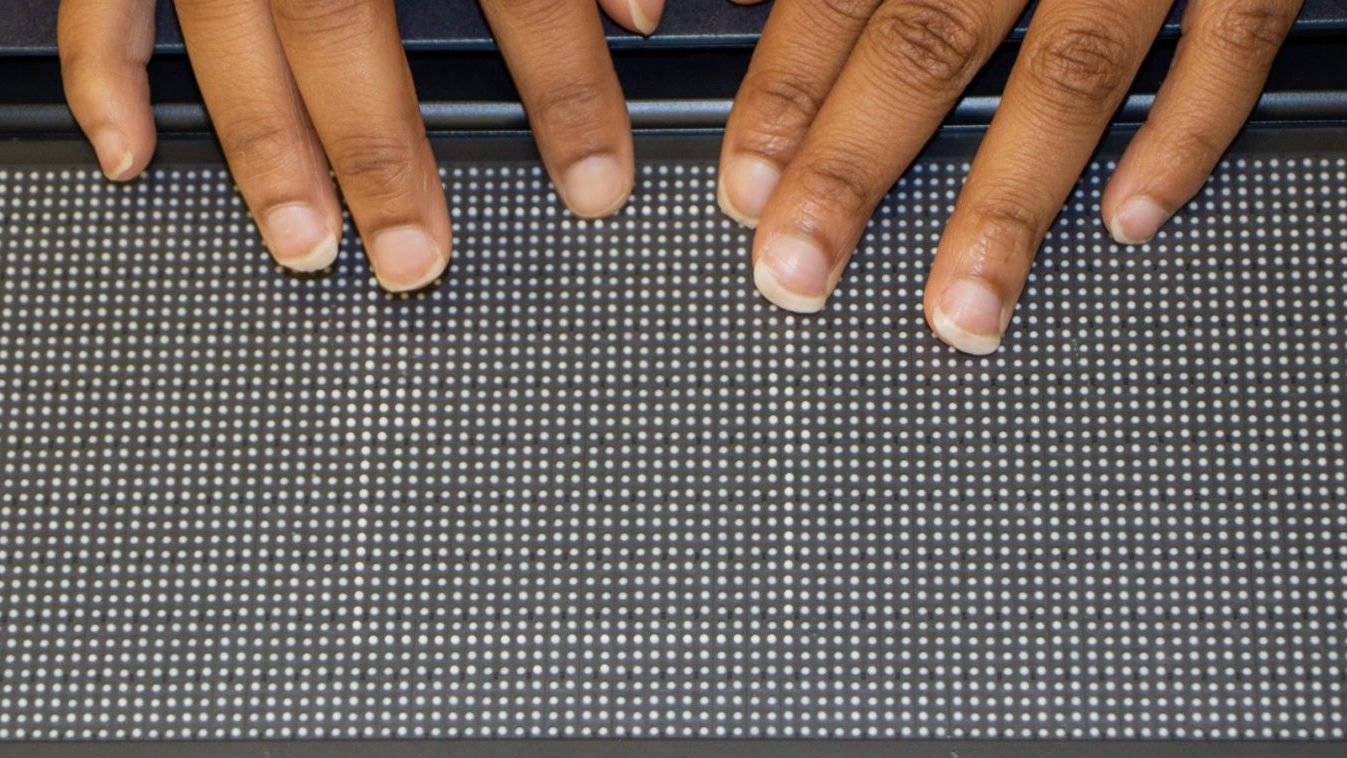This image is an overhead photograph of a black vent or screen with numerous small white circular holes, arrayed across a dark gray background. The vent features intricate detailing with alternating light and dark gray lines framing its edges, transitioning into a black border. Near the top of the image, a pair of dark-skinned fingers, likely belonging to a child, lightly rest upon a piece of plastic above the vent. These fingers, characterized by their short, neatly trimmed, and very round fingernails, create a clear contrast with the vent's pattern. The screen occupies most of the image, and below it, a white table can be seen through the small circular apertures.